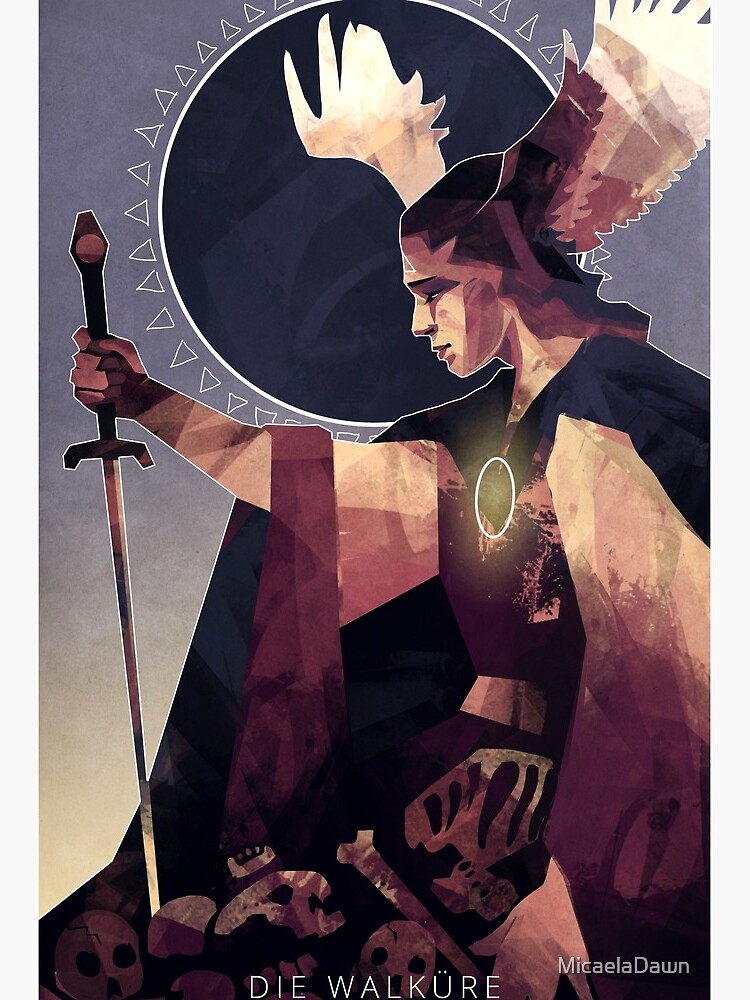The image is a detailed digital art piece resembling a poster featuring a warrior figure. Central to the image is a man, kneeling or seated on his feet, looking to the left. He grips a downward-facing sword, which is embedded into the ground, littered with skulls and bone fragments. The man is attired in a white cape with cranberry accents and a flowing bell-sleeved tunic, also draped in cranberry-colored fabric. Wrapped around his waist is a golden sash, and a glowing, silver orb is positioned at the center of his chest. Notably, he has bird-like wings sprouting from the sides of his head, one of which is illuminated against the dark backdrop.
 
This backdrop consists of a large black circle encircled by white triangles, giving a sun-like appearance, and conveying a layered, almost papery aesthetic. The color palette includes dark and light brown, black, and gold tones. At the bottom of the image are the words "DIE WALKÜRE" in white letters, and in the bottom right corner is the name Michaela Dawn. This intricate composition merges elements of fantasy and warrior iconography, highlighted by its rich details and symbolic elements.